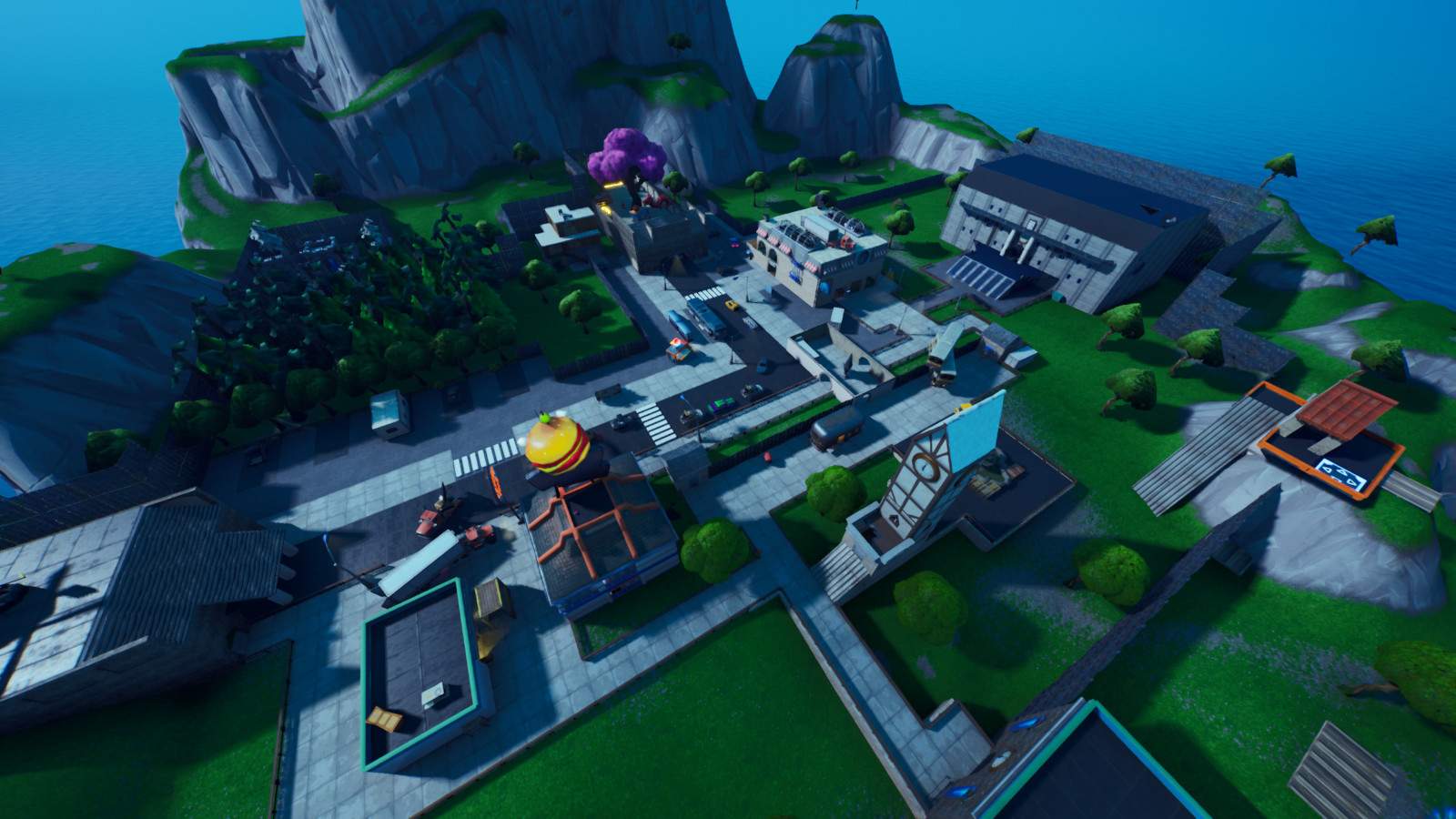This is a vividly detailed digital image resembling a scene from a video game, possibly for platforms like a computer or Xbox. The image is an aerial view, horizontally rectangular in format, with no specific borders. The predominant feature is a turquoise-blue sky occupying the upper portion, contrasting against a blend of natural and man-made elements below. 

In the upper section of the image, rock formations with flat green-topped areas rise prominently. Below these formations, lush green grass spreads across the landscape, divided into neat rectangular sections resembling lawns. The ground level is dotted with numerous trees, some of which are triangular in shape.

A variety of buildings are scattered throughout the scene, primarily to the center and right of the image. There are several white buildings with both peaked and flat roofs, including a tall clock tower with a blue roof situated at the center-right. Toward the far right, there is a striking brown building next to what appears to be ocean waves. Additionally, on the middle right, another prominent building features a triangular roof. Notably absent from the scene are people and vehicles, reinforcing the digital, game-like quality of the image.